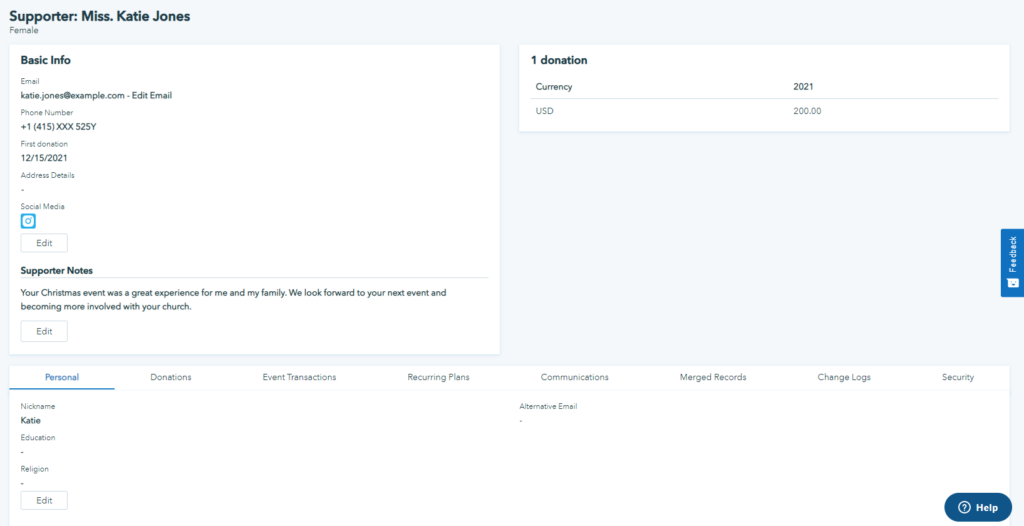The image features a light gray background with detailed information about a supporter named Katie Jones in the top left corner. At the top, the label "Supporter: Miss Katie Jones (Female)" is prominently displayed. Below this label, a white box is divided into several sections containing her basic contact information. 

In the "Basic Info" section:
- Email: katie.jones@example.com (with an option to edit the email)
- Phone Number: +1 (415) XXX-525Y

Further down, there are fields for "First Donation," which is recorded as 12/15/2021, and "Address Details" which appear to be blank. 

Next is the "Social Media" section, which has no entries, followed by an edit button presumably allowing for the addition or modification of information.

In the "Supporter Notes" section, there is a personal comment from Katie: "Your Christmas event was a great experience for me and my family. We look forward to your next event and becoming more involved with your church."

On the upper right side of the frame, it indicates that Katie has made one donation in 2021, amounting to $200 USD. 

Below this financial summary, there are several labels categorizing types of transactions and plans including: "Personal Donation," "Event Transaction," "Recurring Plan," "Communication," and "Merge Records."